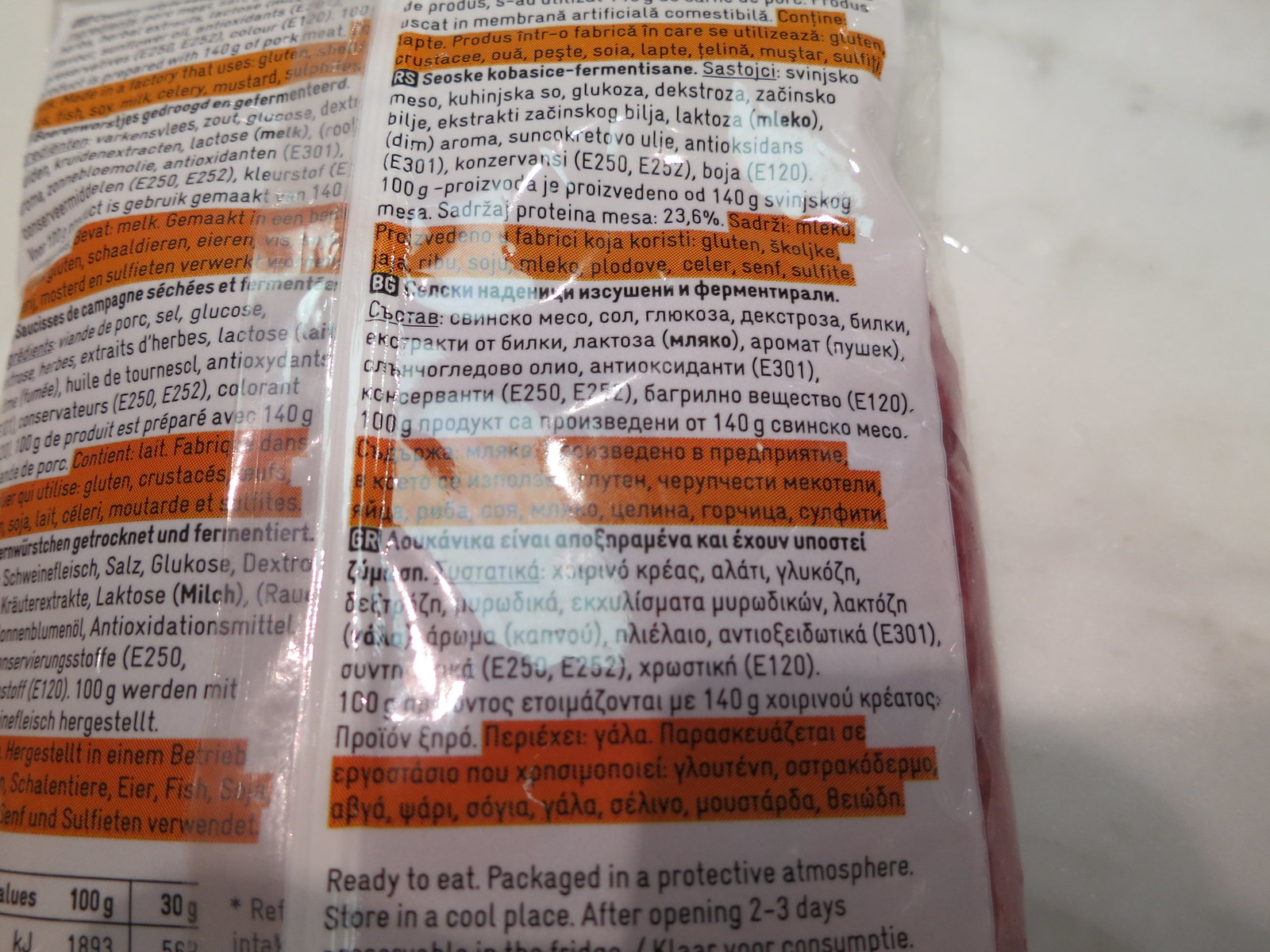The photograph features the back of a thin plastic package, likely containing a food product. The back of the package displays various ingredient lists organized into sections by different languages, all written in black text. Some of these sections are accented with orange highlights. Towards the bottom of the package, a label in English reads: "Ready to eat. Packaged in a protective atmosphere. Store in a cool place after opening. Use within two to three days." However, part of this text is cut off. The package is set on a white marble or stone countertop, which could also be the surface of a table.